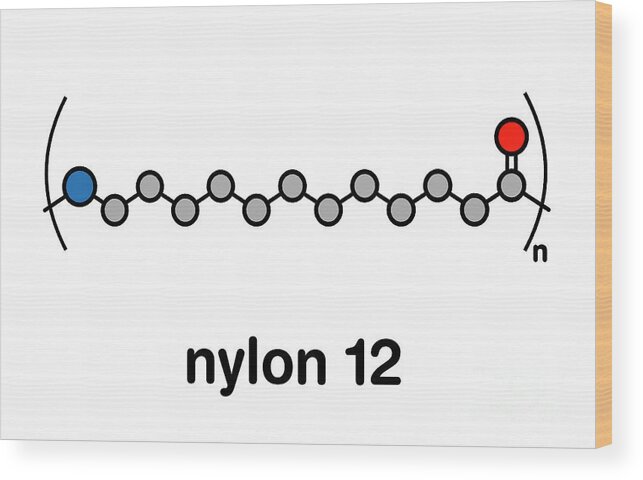The image depicts a detailed illustration of the chemical compound for nylon 12 on a rectangular wooden plaque with a white painted front and natural wood-colored sides. The compound's name, "nylon 12," is labeled at the bottom. Above the label, there is a scientific illustration framed by parentheses, showing a sequence of 14 interconnected circles, each representing atoms. The sequence starts with a larger blue circle on the far left, followed by 12 smaller gray circles, and ends with a red circle on the far right. These circles are connected by short lines, forming a zigzag pattern. To the right of the closing parenthesis is a lowercase "n," likely indicating a functional group or notation relevant to the chemical structure. The entire image features subtle shadowing on the right and bottom, enhancing the three-dimensional appearance of the illustration on the plaque.